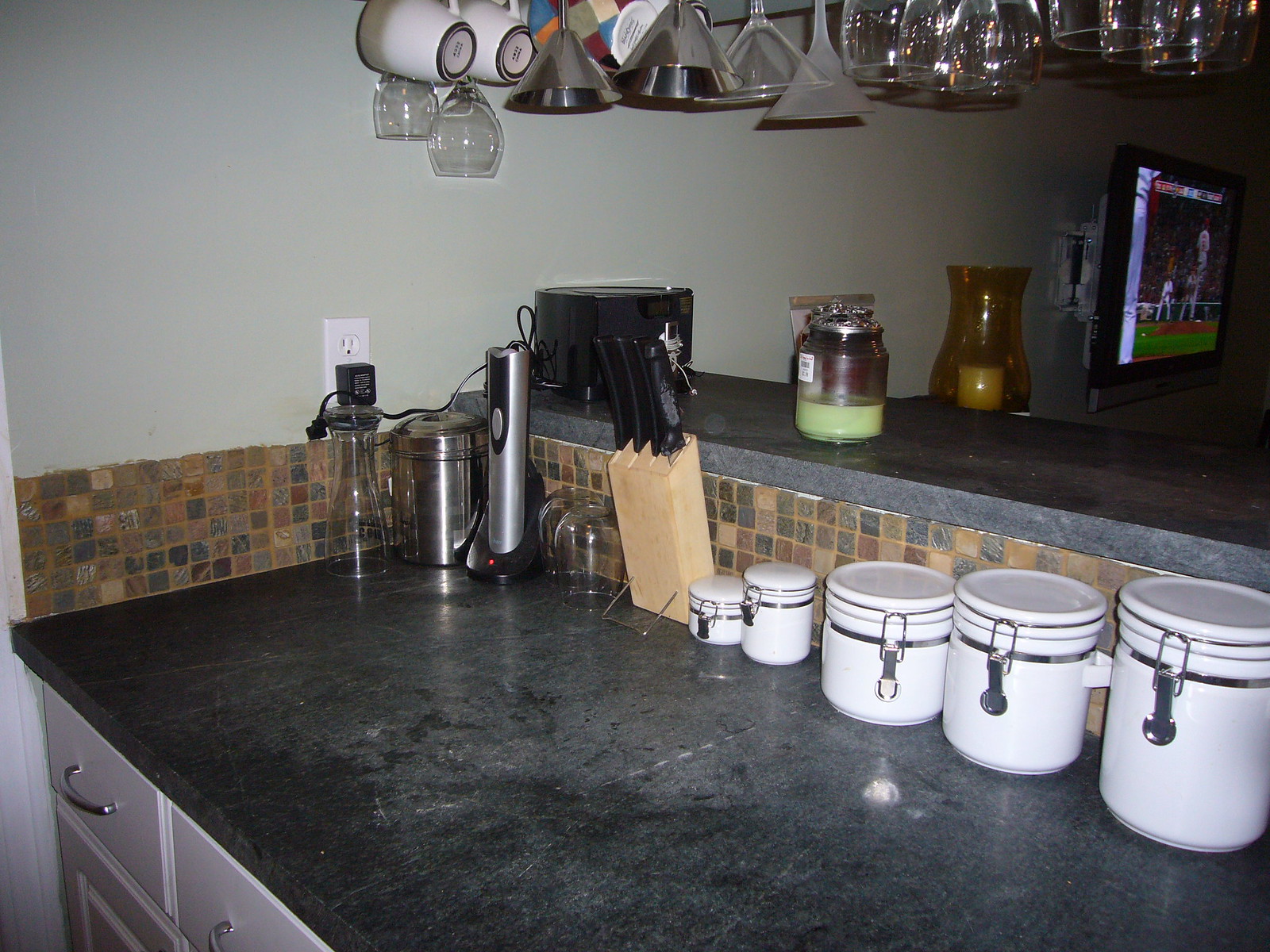A carefully organized and stylish kitchen surface features five white canisters of varying sizes, each adorned with sleek silver locking mechanisms. These canisters, ranging from small to large, are neatly stationed on a low gray countertop. The counter is complemented by a brown, blue, and beige tiled backsplash that adds a touch of colorful elegance to the setting. Adding to the functionality, a knife block is positioned nearby, containing three or four knives. Above the counter, white cabinets with silver handles provide additional storage. Adjacent to the lower countertop is a slightly elevated smaller counter, which holds a candle, among other small items. In the distant background, a TV screen displays a sports game, completing the lively and detailed scene of this modern kitchen.